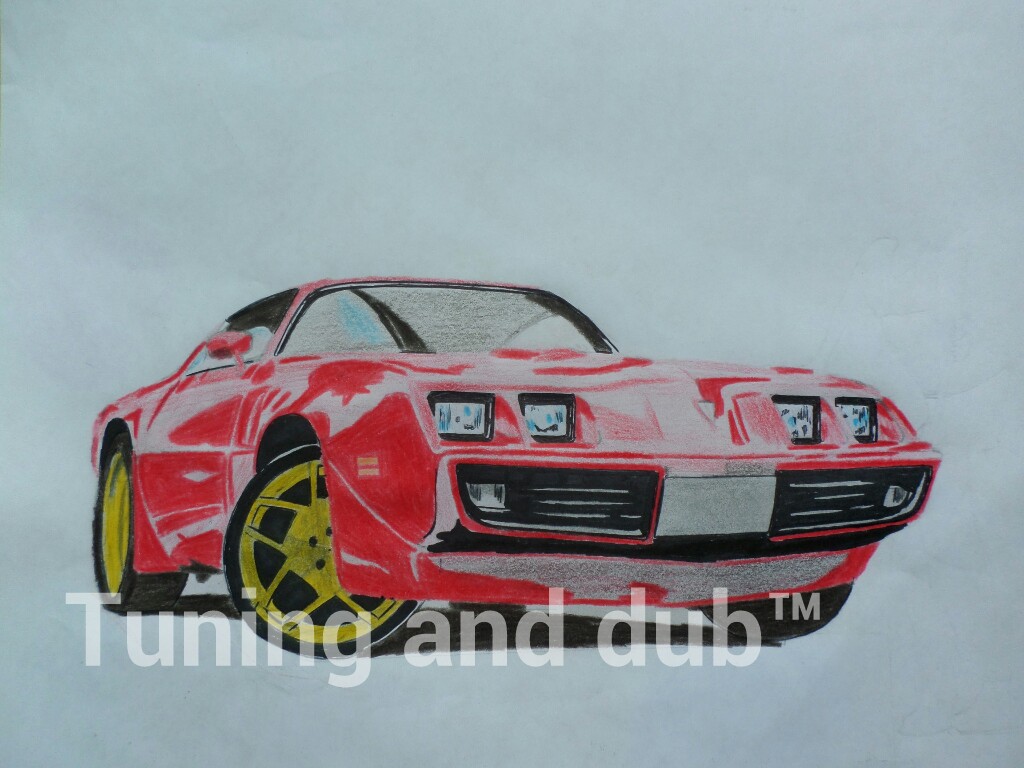The image depicts a detailed drawing of a classic muscle car captured from a low angle, creating a dramatic perspective that emphasizes the vehicle's powerful stance. The car's body is painted a striking red, and only the front and passenger side are visible due to the upward angle of the drawing. The front grille features two square headlights on each side, making a total of four, adding to the car's vintage appeal. The wheels have striking yellow rims and are fitted with thin rubber tires, further highlighting the car's distinctive and stylish design.